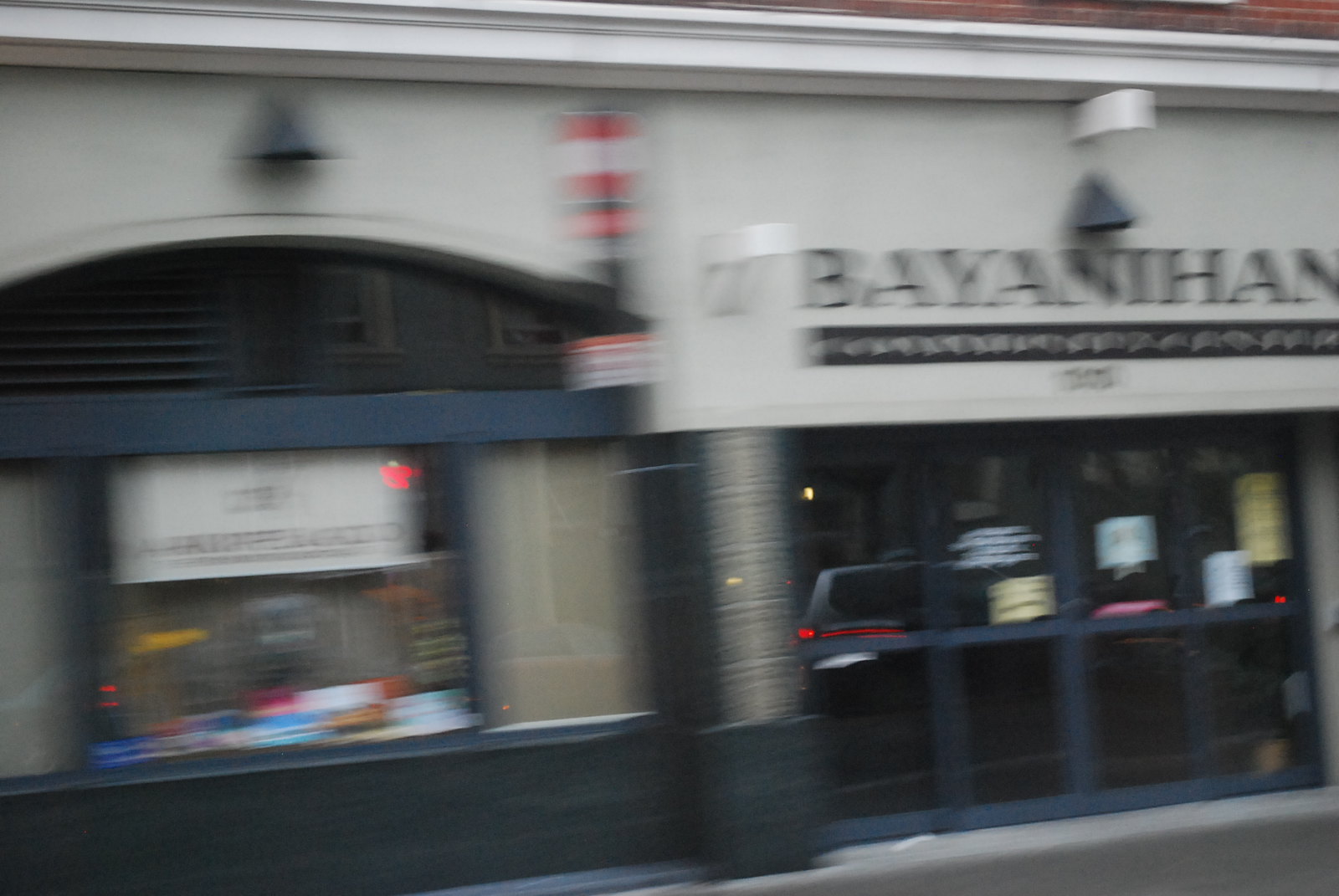The photograph captures a storefront taken from an exterior street view, likely from a moving vehicle, as indicated by the significant motion blur that renders the image extremely out of focus. The establishment's building features distinctive layered architecture: the upper part is constructed of brick, transitioning to an off-white stone section below, and the bottom portion below that is painted a dark greenish-blue color. To the left side of the image, there's a window with a black frame, housing some indistinct red and blue items and a blurry, illegible sign. The lower right-hand corner showcases glass doors, above which "Bayanthan" is written in black letters. Beneath this text, there are additional smaller characters that cannot be made out due to the image's poor clarity. Adding to the storefront’s exterior details are black sconces flanking possibly the entire structure, contributing to its aesthetic. There may be multiple storefronts visible, but the primary focus is the one described.